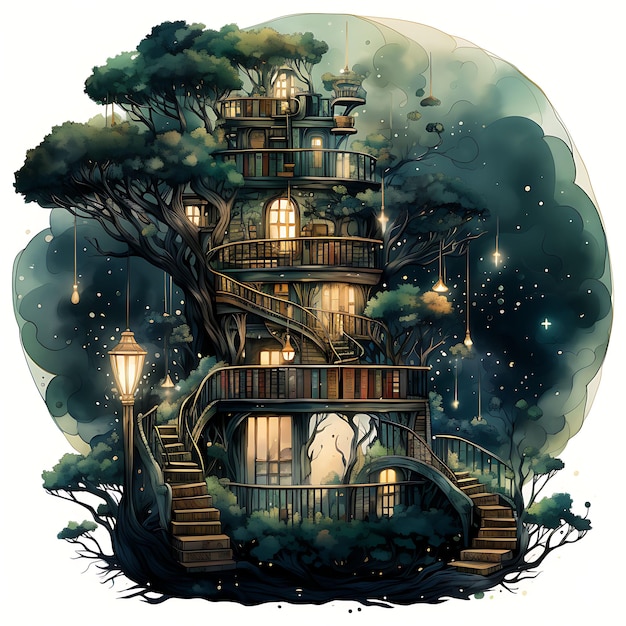This image is a detailed fantasy illustration depicting a magical, multi-storied treehouse that appears to merge nature with whimsical architecture. The scene is dominated by a tall, round-shaped building that ascends four to five stories, each progressively smaller, giving it a towering presence. The structure seems to be crafted from books and wood, featuring brown spiral staircases and railings that wrap around each level. Lanterns and lights illuminate the windows, casting a warm glow against the dark, nighttime sky filled with stars. The house is ensconced in a massive tree, its trunk and branches stretching outward, adorned with lush green leaves and shrubs at the base. Alongside traditional elements, the treehouse radiates a childlike, fairy-tale charm, evoking a sense of adventure and imagination. Earthy tones of greens, browns, and blacks accentuate the illustration's magical theme, while an old-style street lamp adds to the enchanting atmosphere. The entire scene feels both surreal and inviting, emphasizing a world where reading and nature intertwine to take the viewer to another place.